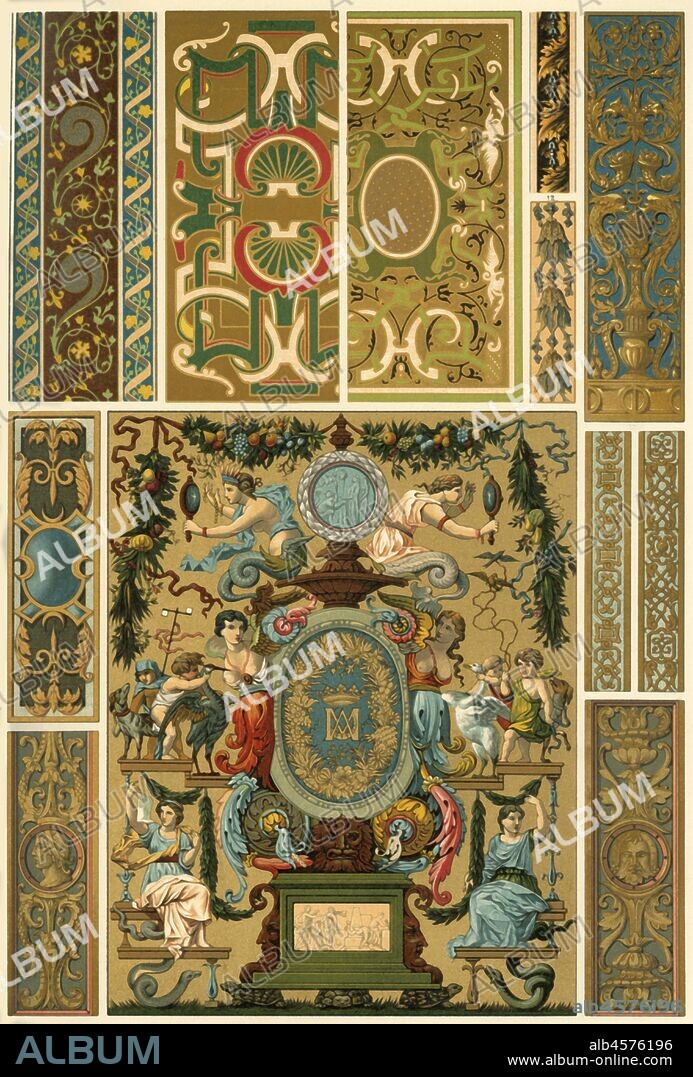The image is a detailed collage with a rectangular, banner-like shape. It is bordered by an ivory-white edge, which also separates the various designs within. The overall background is tan, and there are multiple ornate, golden scroll designs with blue, red, and green backgrounds. Geometric patterns are interspersed throughout, with beige backdrops and golden centers.

At the center of the image is an intricate scene resembling the front cover of an old book. This scene features a red fountain, a green emblem with a golden leaf, and numerous figures, including women holding mirrors, angels, and children. Some women are depicted in robes, interacting with elements like swans and greenery, evoking an old-fashioned, almost biblical atmosphere. Alongside these figures are geometric patterns with a vintage aesthetic.

Semi-transparent white text reading "ALBUM" runs diagonally across the image. At the bottom, a black rectangular banner stretches horizontally, displaying the text "ALB4576196" and "www.album-online.com" in white. This banner reinforces the album theme suggested by the repeated text throughout the collage.